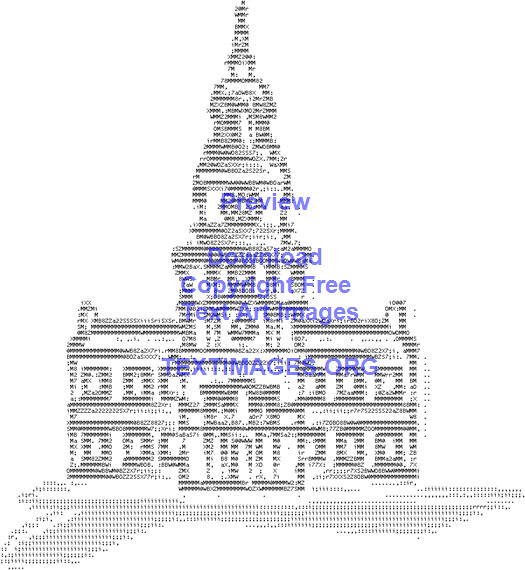This image from textimages.org showcases an intricate piece of text art depicting a large, detailed architectural structure resembling a clock tower or a royal governmental building. The artwork is meticulously crafted using black and white text characters, creating a highly detailed image. The central structure features multiple levels, with a prominent front façade that extends outward, flanked by three windows on each side. Above the façade rises a bell tower topped with a conical roof and a sphere, giving it a majestic appearance. The background is white, further highlighting the detailed design. The blueprint-like quality of the image suggests precision, indicative of what a computer might generate. The image includes text in blue in the foreground that reads "Preview, Download, Copyright Free, Text Art Images, textimages.org," emphasizing its source and the nature of its availability.